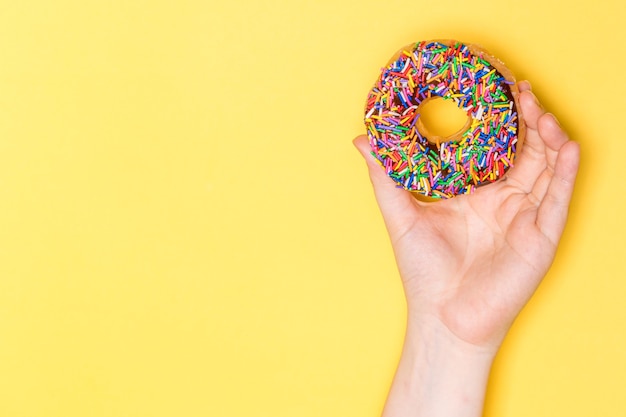The image depicts a horizontal scene with a bright yellow background entirely devoid of text or other objects. Positioned towards the right side of the frame, a Caucasian hand—possibly male but indistinctly gendered—holds a donut up to the wrist. The donut, featuring a classic hole in the center, is generously covered in chocolate icing, which is barely visible beneath a dense layer of multicolored sprinkles. These sprinkles are vibrant in hues of red, blue, green, purple, orange, pink, and indigo, giving the donut a rainbow-like appearance. The hand's thumb is positioned on the left side of the donut, with the other fingers curled around the right side, holding it securely in a natural, hooked grasp. The yellow background serves as a stark, uncomplicated backdrop, emphasizing the vivid colors and details of the hand and donut.